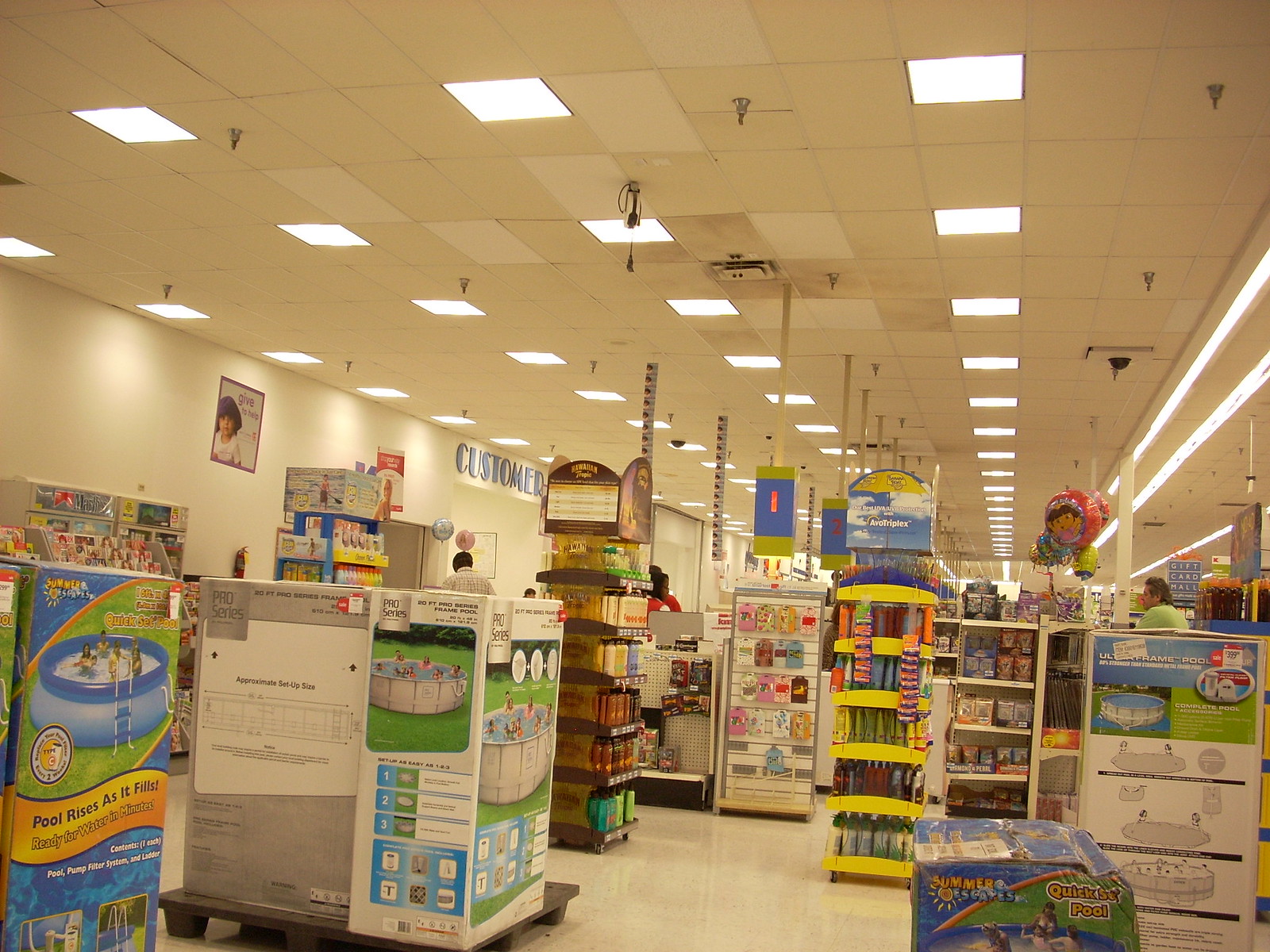A vibrant image captures the bustling ambiance of a large grocery store, possibly a Walmart, distinguished by the characteristic blue and lime green color scheme. In the background, both traditional and self-checkout lanes are visible with staff members and a few customers milling about. Fluorescent lights cast a bright glow over the aisles, ensuring every detail is well-lit. Prominently featured in the sports and seasonal department section, there is a large box advertising a children’s hot tub or swimming pool. Nearby, an eye-catching display case showcases an array of Banana Boat sunscreen products, emphasizing the store's preparedness for sunny weather activities. The scene epitomizes a typical, busy shopping day, capturing the essence of modern retail environments.